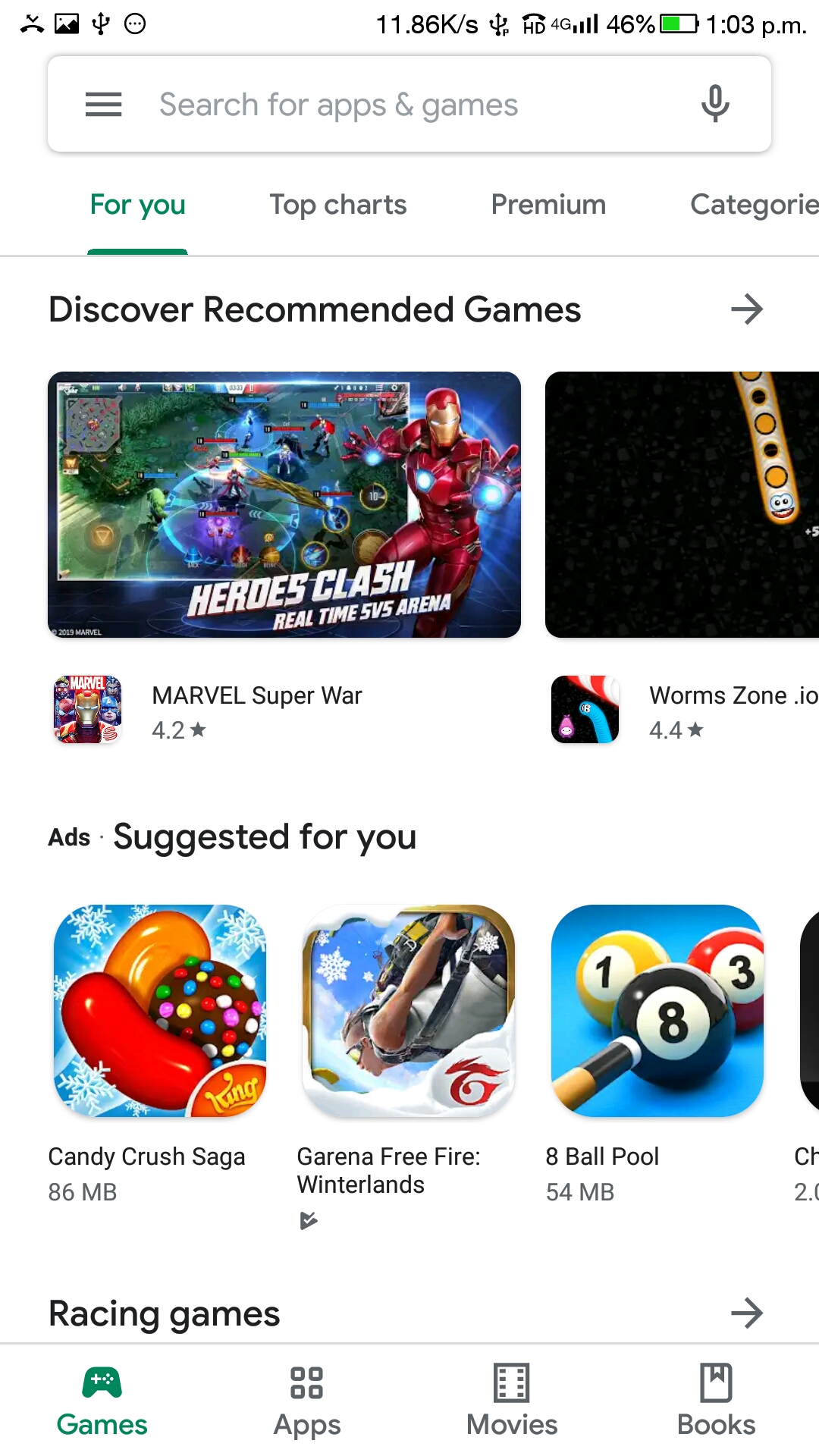This screenshot captures a user's experience on the Google App Store, displayed on a smartphone set to light mode at 1:03 PM, as indicated by the menu bar at the top. The menu bar also reveals a missed call notification, a recent image download, network connection status, and battery level information. 

At the top of the screen, there is a search bar with a microphone icon to the right and a vertical three-bar menu icon to the left, with "Search for apps and games" written inside the search bar.

Below the search bar, a featured section displays the label "Discover recommended games" and includes an advertisement for "Heroes Clash," prominently featuring Iron Man in bright, dynamic gameplay imagery. Next to this ad is "Worms Zone IO," showcased with a darker, more minimalist screenshot that features a long cylinder with dots indicating a gaming level.

Further down, there is a section labeled "Ads suggested for you." This includes an advertisement for "Candy Crush," showing various candies set against a festive winter background, another for "Garena Free Fire Winterlands," depicting a character in mid-skydiving action, and an ad for "8 Ball Pool," displaying a black 8 ball, a yellow 1 ball, and a red 3 ball.

At the bottom of the screen, the user interface features tabs labeled "Games," "Apps," "Movies," and "Books," with a section titled "Racing games" denoted by an arrow pointing to the right, suggesting more selections can be viewed.